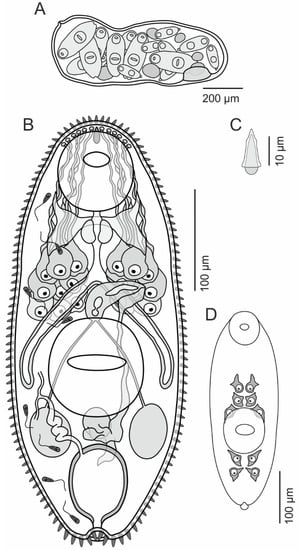This image is a detailed black and white scientific illustration, potentially from a textbook, depicting various stages or types of cells labeled A, B, C, and D. 

In Image A, the depiction resembles an amoeba or a cell, elongated and lumpy with a defined outer wall. Within it, there are several smaller ovals, each containing a nucleus-like structure, along with round items dispersed inside. The size is measured approximately 800 microns long and 300 microns tall, with a scale bar indicating 200 microns.

Image B is a larger, blown-up portrayal of what could be an embryo or a related cellular structure, displaying a complex internal system suggestive of organs or digestive tracts, with several circular and blob-like shapes inside. The illustration features cilia along the outer edge and internal features that might represent kidneys or a digestive system. This cell is about 400 microns long and 200 microns wide, with a scale bar of 100 microns.

Image C represents a much smaller, teardrop-shaped object with a triangular sheath-like structure covering part of it. This image is significantly smaller, approximately 15 microns tall and 5 microns wide, with a scale bar indicating 10 microns.

Finally, Image D shows another oval-shaped structure differing from the others, with two prominent circles positioned at the top and center, and numerous smaller elements dispersed within, giving an impression of having eyes. The structure measures around 400 microns tall and 200 microns wide, with a scale bar of 100 microns. 

Each part of the illustration emphasizes various biological forms, likely representing different cell types or stages of a similar organism.